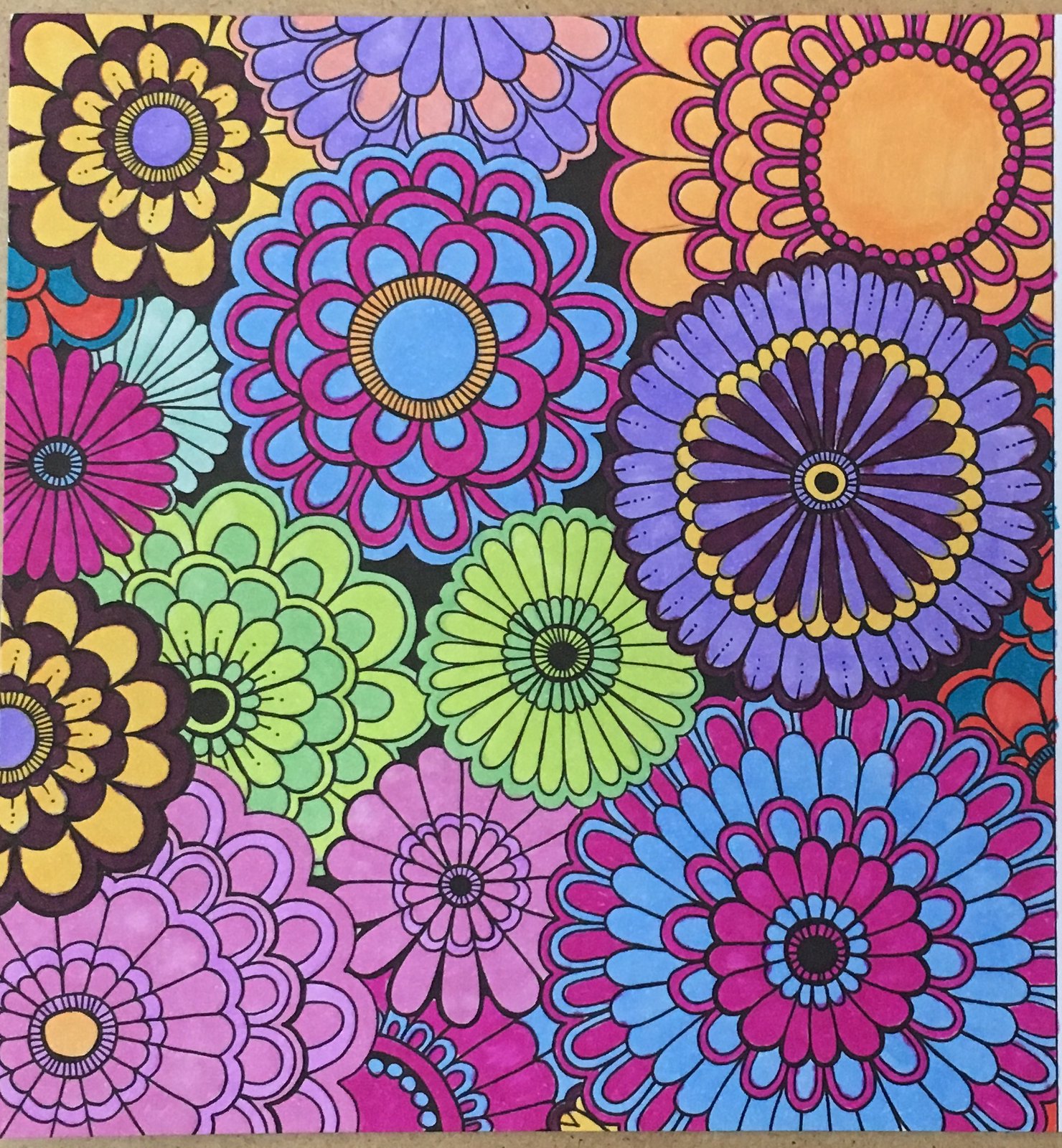The image is a vividly colorful, hand-drawn illustration resembling a mandala from an intricate adult coloring book. It fills the entire frame and appears to have been digitally scanned. The composition is a layered collage of two-dimensional flower faces, viewed top-down without stalks or leaves. Each flower is unique in design and color, showcasing a spectrum of hues including mauve, yellow, green, pink, orange, blue, teal, lavender, and brown. Some flowers have multiple layers of concentric petals, while others feature just one or two rings, with petal shapes ranging from thin and long to short and fat.

In the top left, a flower with a dark chocolate brown border transitions through light orange bands and hash marks, culminating in a purple center. Next to it, a flower alternates between pink and purple outlines and sections. Another nearby flower is outlined in blue and cycles through hot pink and blue with an orange hash mark center. Two simplistic flowers, one olive green and the other hot pink with a black outline, feature hash marks around white rectangles with black centers.

Other distinct flowers include a greenish-blue one transitioning to red, a hot pink and orange flower with a multicolored hot pink circle center, and pink flowers with hot pink borders and yellow centers situated in the lower left. Some flowers used light green and dark green hues, with details like flanked dark and lime green outlines. Though the colors are predominantly within the lines, slight deviations hint at hand-coloring with markers, adding a personal touch to this richly detailed and meticulously executed piece.